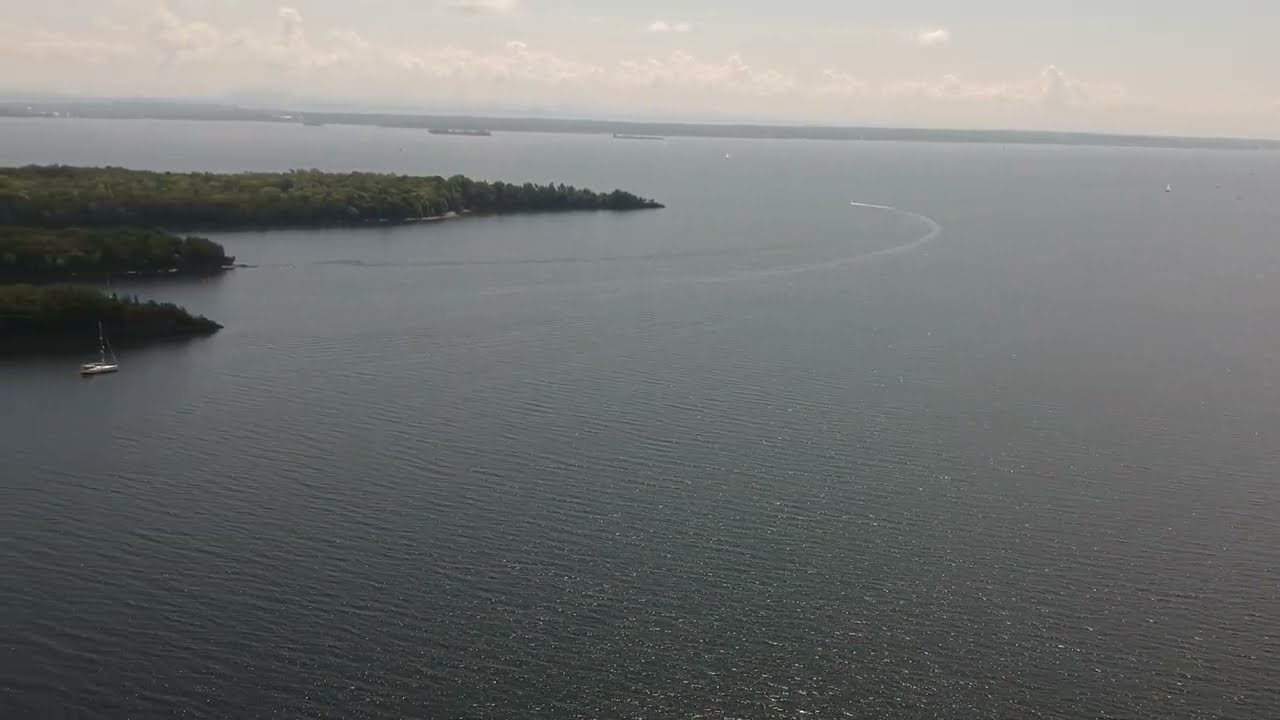The photograph, captured from an aerial perspective during the daytime, depicts a serene landscape with a striking contrast between the elements. The top section of the image features a light gray skyline adorned with a thin stripe of fluffy gray-white clouds stretching across a darker sky. Below the sky, a slim strip of land touches the horizon. Dominating the bottom three-quarters of the image is a vast expanse of still, deep dark blue ocean.

In the upper left portion of the scene, three grassy knolls or inlets extend into the water. The foremost knoll is the smallest, and just in front of it, a sailboat with its sails down can be seen navigating the waters near the longest green inlet. Additionally, there is a faint trace of a motorboat curving around the left side of the inlet, its wake subtly trailing behind.

The land in the upper left part of the image appears as an uninhabited island, covered in greenery without any buildings, marked only by trees and bushy grass. The peaceful composition is characterized by a palette of deep green, brown, ocean blue, white, and gray hues, enhancing the overall tranquility of this extensive landscape scene.